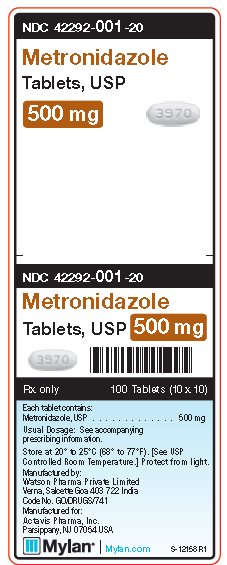The image captures an advertisement or label for Metronidazole Tablets USP. In the upper section, the name "Metronidazole Tablets, USP" is prominently displayed. Beneath this, a brown rectangle showcases the dosage "500 mg". A detailed picture of an oblong, egg-shaped pill marked with the numbers "3970" is prominently featured. 

Moving downwards, there's a clear white space before reaching the bottom area where the label "NDC 42292-001-20" is listed. The drug name "Metronidazole Tablets USP, 500 milligrams" is reiterated. An adjacent area contains a scannable barcode.

Further information is enclosed within a blue square at the bottom, stating: "Each tablet contains Metronidazole USP 500 milligrams. Usual dosage: see accompanying prescribing information." It also includes instructions on storage and other pertinent details.